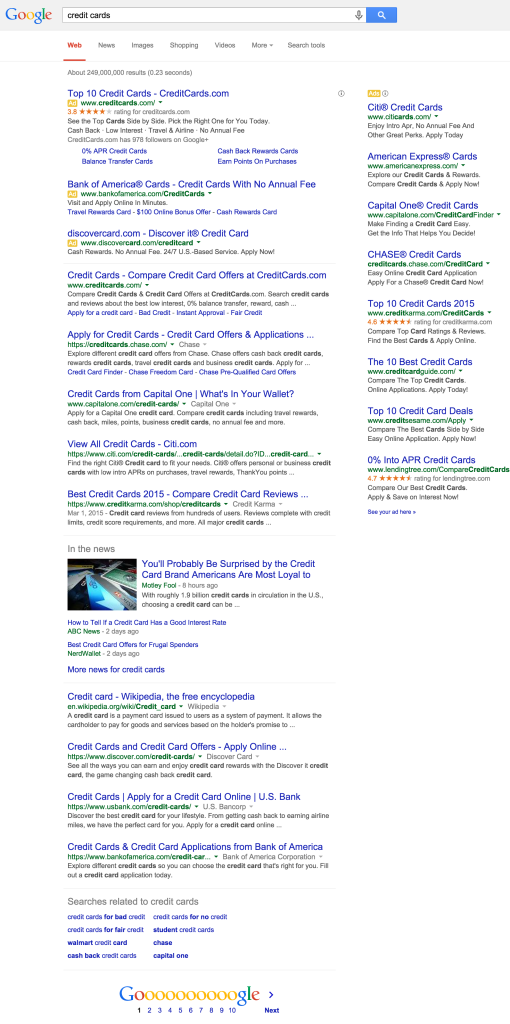A detailed screenshot of a Google search for credit cards, displaying a variety of search results and hyperlinks. At the top of the page, the prominent Google logo signifies the platform. Following this are assorted hyperlinks to various resources related to credit cards. Key links include: "Top 10 Credit Cards," "CreditCards.com," "Bank of America Credit Cards," "Credit Cards with No Annual Fee," "Discover Credit Card," and "Compare Credit Card Offers at CreditCards.com." Other notable results include "Apply for Credit Cards," "Credit Cards for Capital One," "View All Credit Cards at Citi.com," "Best Credit Cards 2015," "Compare Credit Card Reviews," and an intriguing link suggesting, "You'll Probably be Surprised by the Credit Card Brand Americans are Most Loyal To." Additional results provide information on identifying good interest rates in "How to Tell a Credit Card has a Good Interest Rate," general knowledge from "Credit Card - Wikipedia, The Free Encyclopedia," and various links to online credit card applications like "Credit Cards and Credit Offers - Apply Online" and "Credit Cards - Apply for a Credit Card Online with U.S. Bank." On the right side of the page, in smaller font text, there are extra links to other credit card-related websites, providing a comprehensive overview of available credit card options and resources.